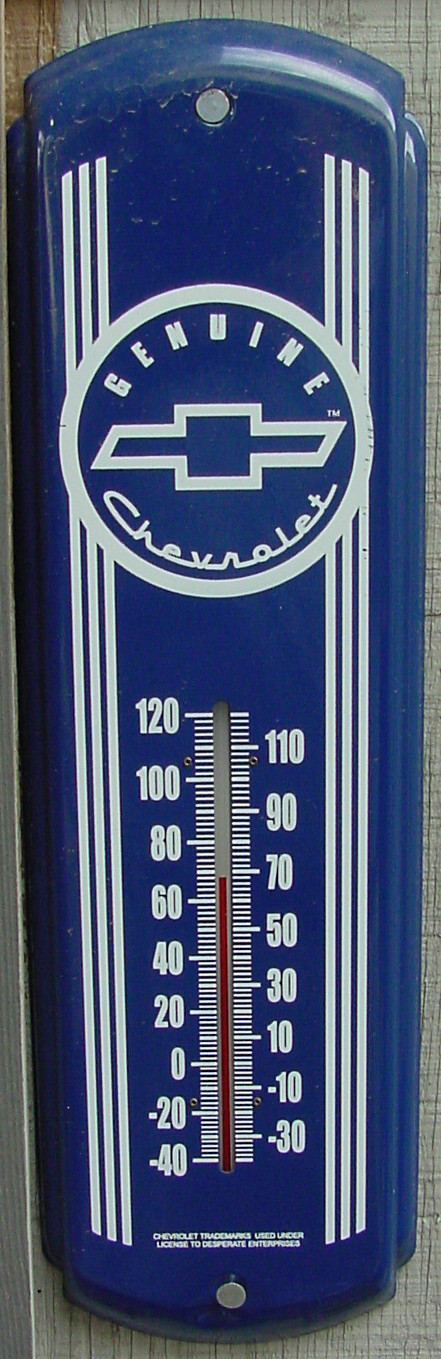The image is a detailed illustration featuring the Genuine Chevrolet logo. Positioned centrally is the iconic Chevrolet emblem – a golden bowtie shape with a square middle. Surrounding the emblem on either side are white lines, creating a symmetrical border. Below the logo, there's a caption stating "Chevrolet trademark is under license to desperate entrepreneur."

The background is predominantly white, and at the bottom, there is an additional golden element adding a touch of elegance to the design. The main feature of the image is a blue thermometer, prominently placed in the center. The thermometer displays temperatures in both Fahrenheit and Celsius, with the left side showing degrees from -40 to 120 in increments of 20, and the right side showing degrees from -30 to 110 in increments of 20. The current temperature reading on the thermometer shows approximately 69 degrees, indicated by a red marker.